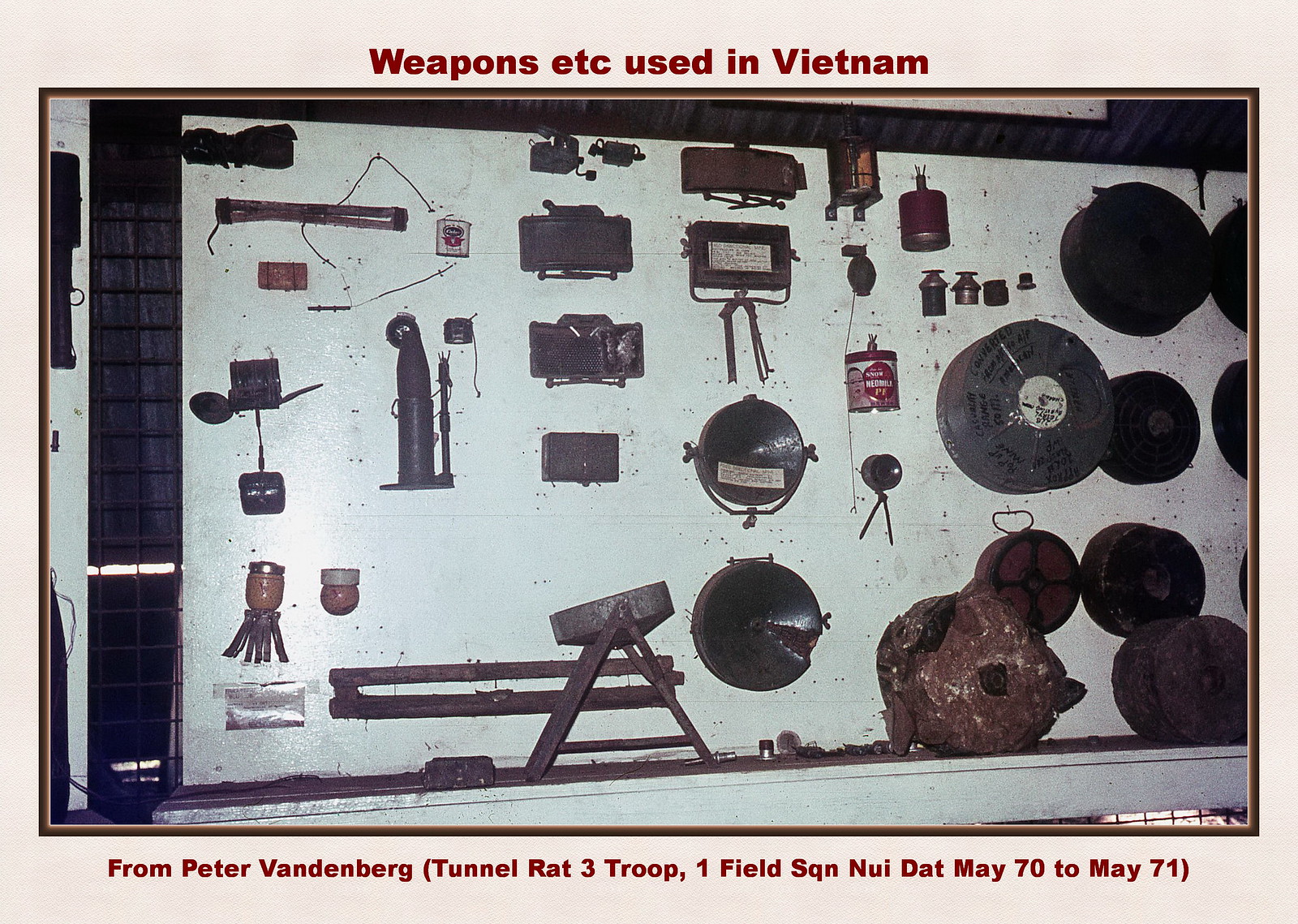This image captures a meticulously organized display case housing a variety of metal objects used during the Vietnam War. The photograph is bordered in white, with an inscription at the top that reads "Weapons, etc. used in Vietnam" rendered in brown text, and at the bottom, "From Peter Vandenberg, Tunnel Rat 3 Troop, 1 Field SQN, Nui Dat, May 1970 to May 1971." The objects, likely a collection of weapons and explosive devices, include items resembling landmines, grenades, claymore mines, and other small explosives, displayed against what appears to be a white wall. The array is arranged in a loose grid pattern, showcasing the variety of tools and devices used by military personnel during the conflict. Though the exact nature of some items might be unclear to non-military viewers, the display evidences the diverse and potentially deadly arsenal that characterized the Vietnam War.